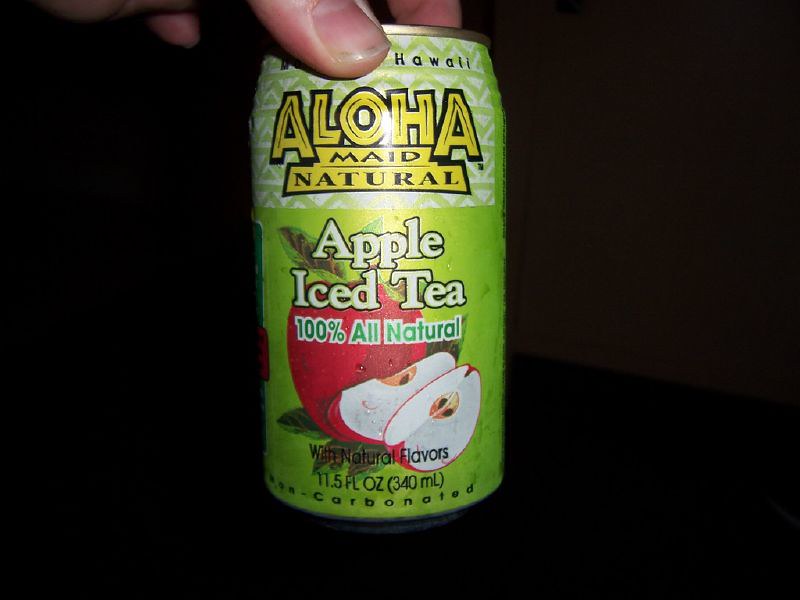The image depicts a person's left hand, slightly dirty under the thumbnail, holding a predominantly light green can of Apple Iced Tea. The can is marked with the brand "Aloha Maid Natural," with "Maid" spelled as "MAID." At the top of the can, written in yellow against a triangular green pattern on a white background, are the words "Aloha Maid Natural." Beneath it, "Apple Iced Tea" is displayed in white letters, outlined in black, followed by "100% All Natural" in green letters with a white outline. The next section features an image of a whole red apple and two apple slices showing their white flesh and brown seeds. Towards the bottom of the can, it states "With Natural Flavors," "11.5 fluid ounces (340 milliliters)," and "Non-carbonated" in black letters. The can is held against a black background.